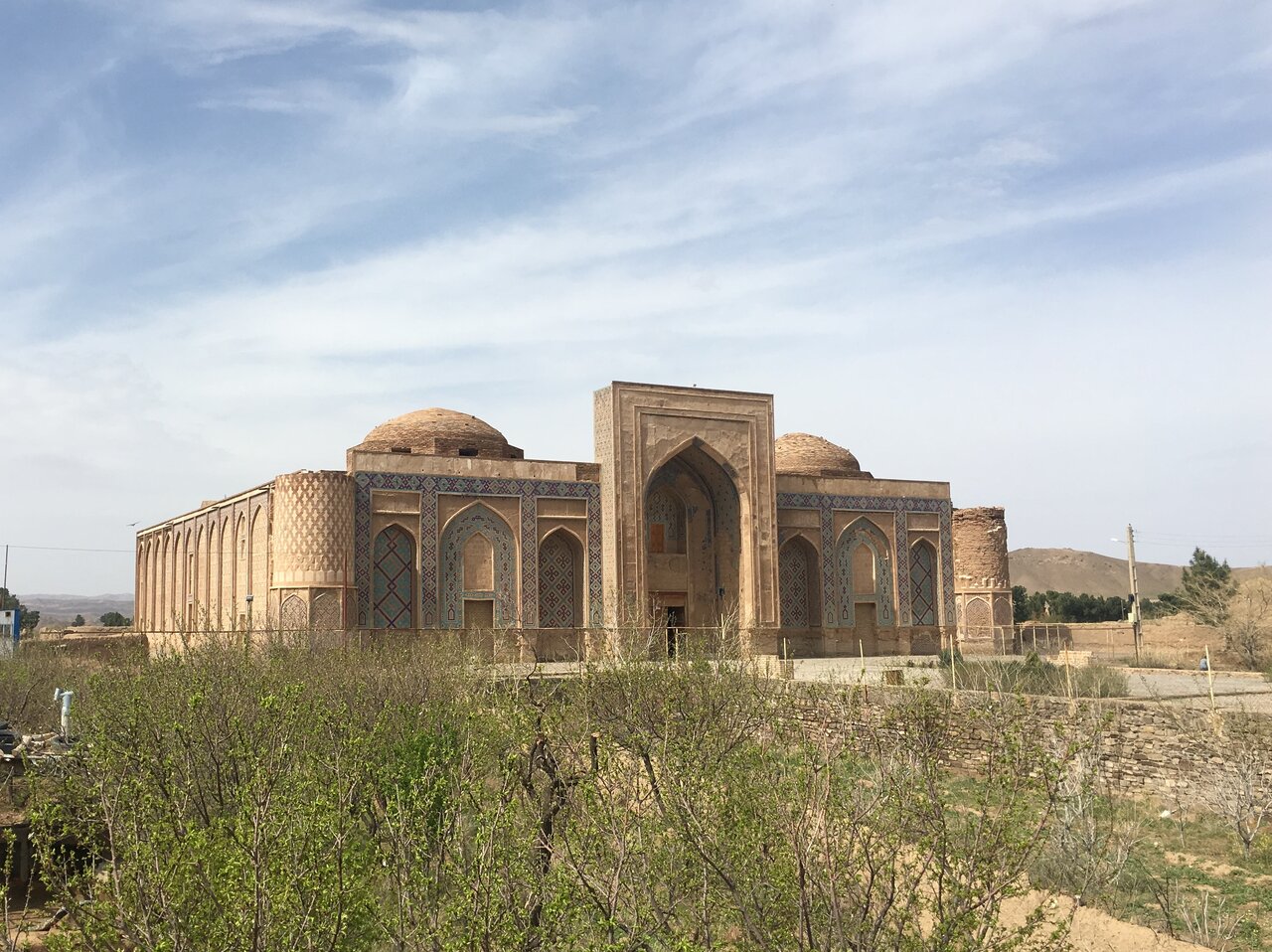The photograph captures a striking Middle Eastern or possibly South Asian building, characterized by its grandiose Middle Eastern-inspired architecture. The structure features two prominent dome-shaped structures on the roof and a colossal arched entrance that is taller than the building itself. The front façade is adorned with six windows—three on each side of the entrance—all topped with curved domes, typical of this architectural style. Captured from approximately 60 feet away, desert brush and a garden featuring sparse shrubbery are visible in the immediate foreground, suggesting an autumn or winter setting. Additionally, a water pump and a valve, possibly for farming, can be seen near the building. Surrounding the temple-like building are power lines and telephone poles, set against a backdrop of hills or mountains. The skies are partly overcast, casting shadows that indicate the sun is positioned to the left of the image. This blend of features suggests the building could be in a Middle Eastern, South Asian country, or even a specific region in the United States.